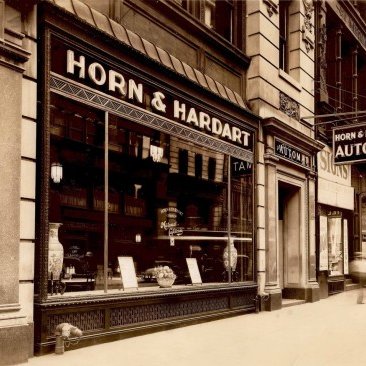This is a black and white, possibly sepia-toned, vintage photograph of a famous early 20th-century restaurant storefront, Horn & Hardart. The image captures a portion of at least a two-story building, though the top is cut off. The photo is taken at a three-quarter angle facing right, revealing a flat facade with a large, three-pane picture window at its center. Above the window, a prominent black horizontal sign displays "HORN & HARDART" in bold white capital letters. 

Behind the window, the restaurant's interior includes a counter adorned with a central basket of flowers flanked by vases on either side, and two smaller signs on either side of the basket. To the right of the window, a doorway featuring a white sign above it leads into the establishment. At street level, the storefront meets the cement sidewalk with a brick base. To the left, a stone wall and, just above it, residential windows suggest apartments above the store. Adjacent to the restaurant is another building with an ornate doorway typical of early 1900s architecture, though its name is unclear. Additionally, there is a sign for Horn & Hardart projecting out over the front door, further identifying the iconic eatery.